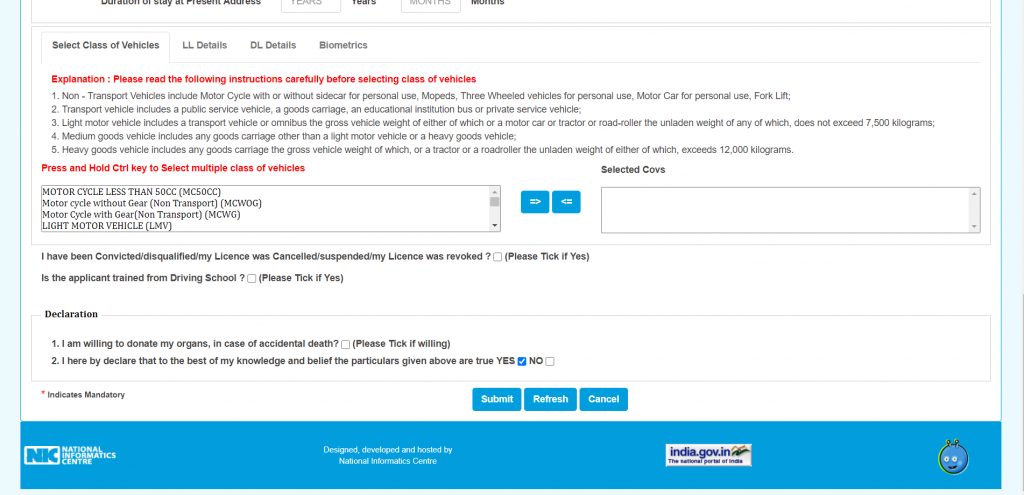### Detailed Caption:

The image is a screenshot displaying a user interface with a clean, white background. At the top of the interface, there are multiple tabs listed as "Select Class," "The Vehicles," "LL Details," "DL Details," and "Biometrics." Beneath these tabs, an explanatory note is prominently highlighted in red, stating: "Please read the following instructions carefully before selecting the class of vehicles."

Following this note, instructions are provided in a numbered list:
1. Non-transport vehicles include motorcycles with or without a sidecar for personal use, three-wheeled vehicles for personal use, motorcars for personal use, and forklifts.
2. (Further instructions continue from points two to five, though not fully visible or detailed in the provided text.)

Additionally, another instruction in red informs users to "Press and hold the CTRL key to select multiple classes of vehicles."

Below this, the interface is divided into two main selection boxes. The first box, labelled "Selected Codes," is currently empty. The second box includes an option for "Motorcycle less than 50cc" with the code "MC50cc" indicated in parentheses.

At the bottom center of the interface, three buttons are visible: "Submit," "Refresh," and "Cancel," offering options for the user to proceed, reload, or exit the selection process.

Overall, the interface appears to be designed for selecting specific classes of vehicles with detailed instructions and multiple interactive elements.